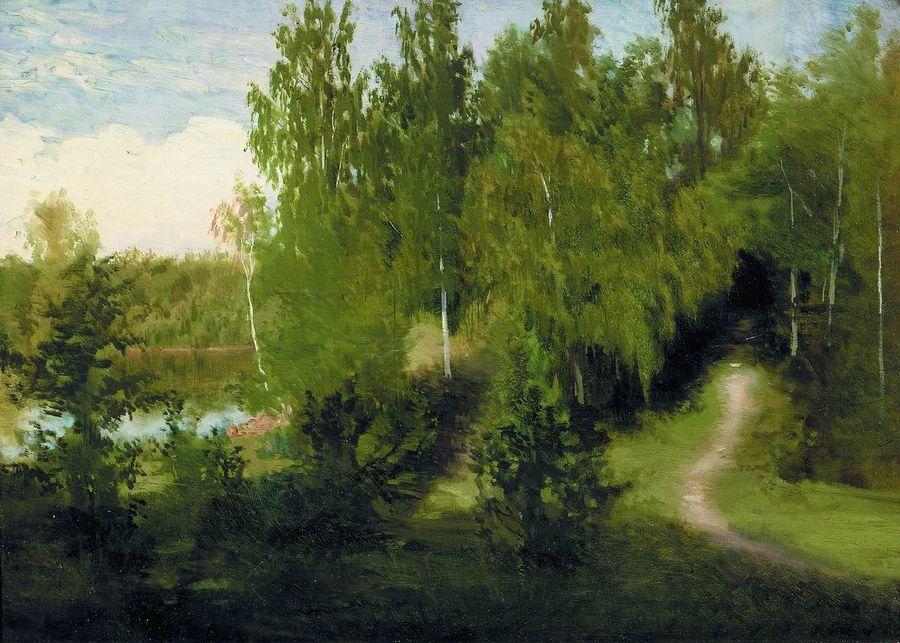The painting depicts a lush, verdant landscape dominated by various shades of green. The foreground features a meandering dirt path that appears gray in color, flanked on either side by short, bright green saplings and tall trees with thin white trunks, possibly birch. This path winds its way into a dense tree line that stretches from right to left. To the left of the path lies a small, reflective body of water that mirrors the surrounding greenery. Around this lake area, more trees and grassy banks can be seen. The sky above is a serene powder blue, adorned with fluffy white clouds, adding a tranquil backdrop to the vibrant foliage below. Dark shadows and additional plant life, with their darker green hues, occupy the foreground, enhancing the depth and richness of the scene. This painting’s exquisite detail captures the beauty of nature through its vivid green trees, the calm water to the left, and the inviting path leading into the densely forested area.